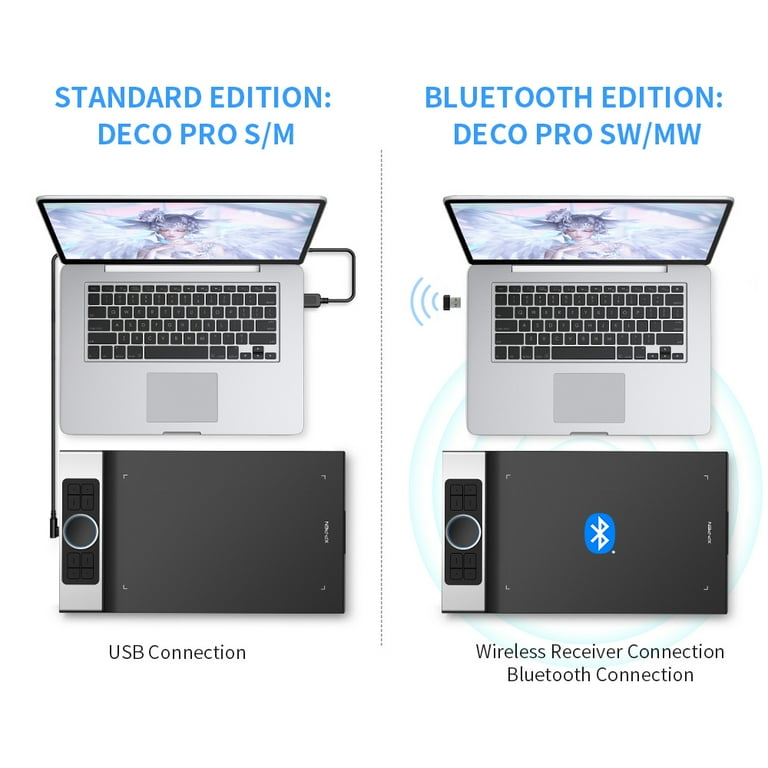The image is a detailed comparison of two connection methods for the Deco Pro drawing tablet when used with a laptop. Both sides of the image feature an idealized aerial view of the same black and silver laptop with a woman's image and a multicolored background on the screen. 

On the left, labeled "Standard Edition: Deco Pro S/M," the laptop is connected to a drawing tablet via a USB-A cable. The tablet, positioned below the laptop, is a flat, rectangular device with a large black area and a silver section that includes a black segment with a circular hole. "USB Connection" is noted at the bottom.

The right side, labeled "Bluetooth Edition: Deco Pro SW/MW," shows the same laptop with a wireless connection. A Bluetooth dongle, represented with signal arcs, is positioned near a USB port on the laptop, indicating the absence of a physical cable. The drawing tablet below now features a Bluetooth logo in the center of its black area. The bottom text reads "Wireless Receiver Connection, Bluetooth Connection."

This comparison highlights the difference between the USB and Bluetooth connection options for the Deco Pro drawing tablet.